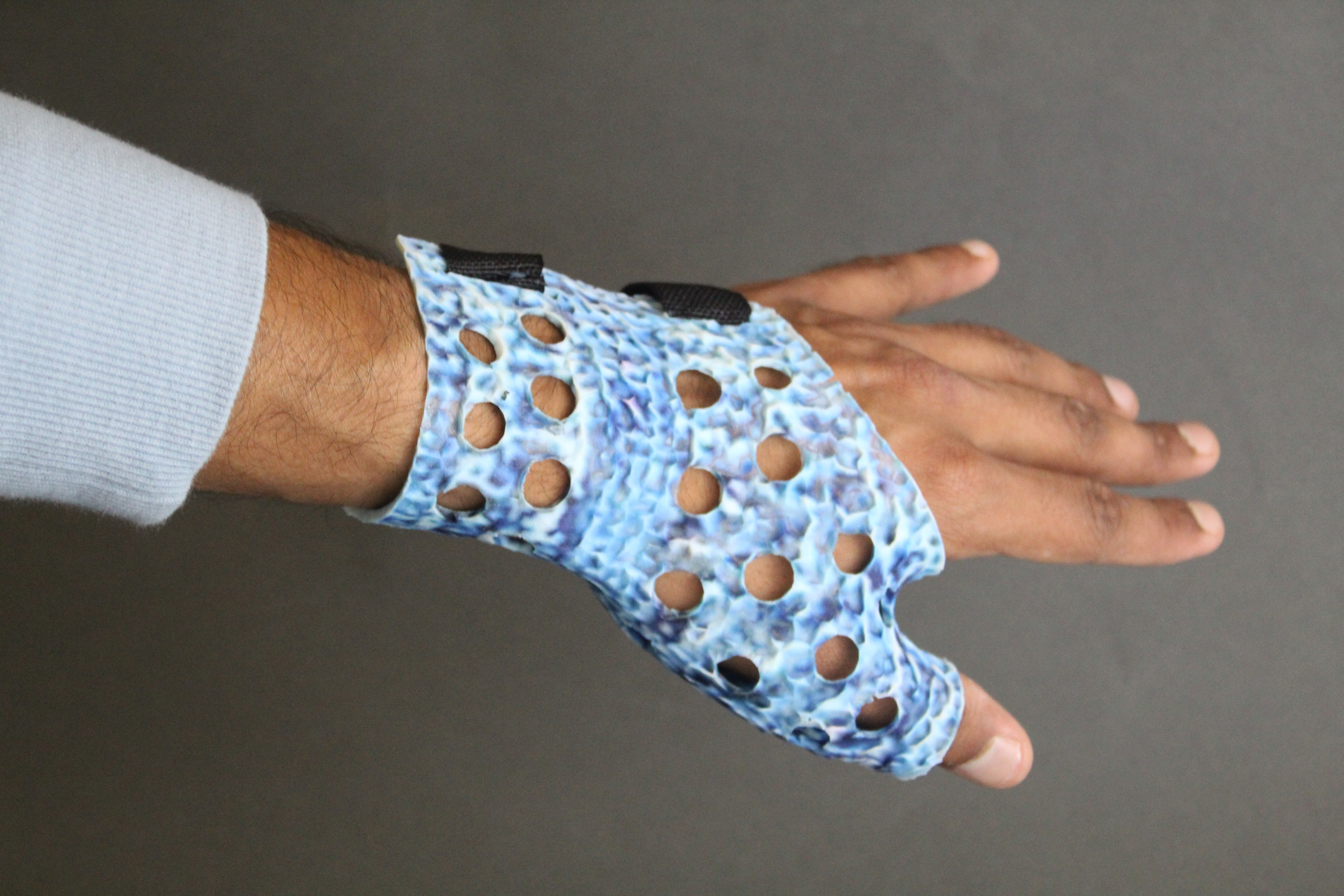The image depicts a close-up of a man's hand, possibly of Asian or Black descent, positioned prominently against a grayish-tan background. His arm, visible from the left, reveals a gray sweater with the sleeve slightly pulled up. The focus is on a distinctive blue and white brace or glove worn over the hand. This glove, characterized by numerous ventilation holes, covers most of the hand, extending to the knuckles and partially around the thumb. It appears to be held together by black fasteners, likely velcro or buckles, visible near the top edge. The device might serve various functions, potentially for improving grip or support, similar to equipment used by drummers and singers to enhance hand stability and prevent slippage.